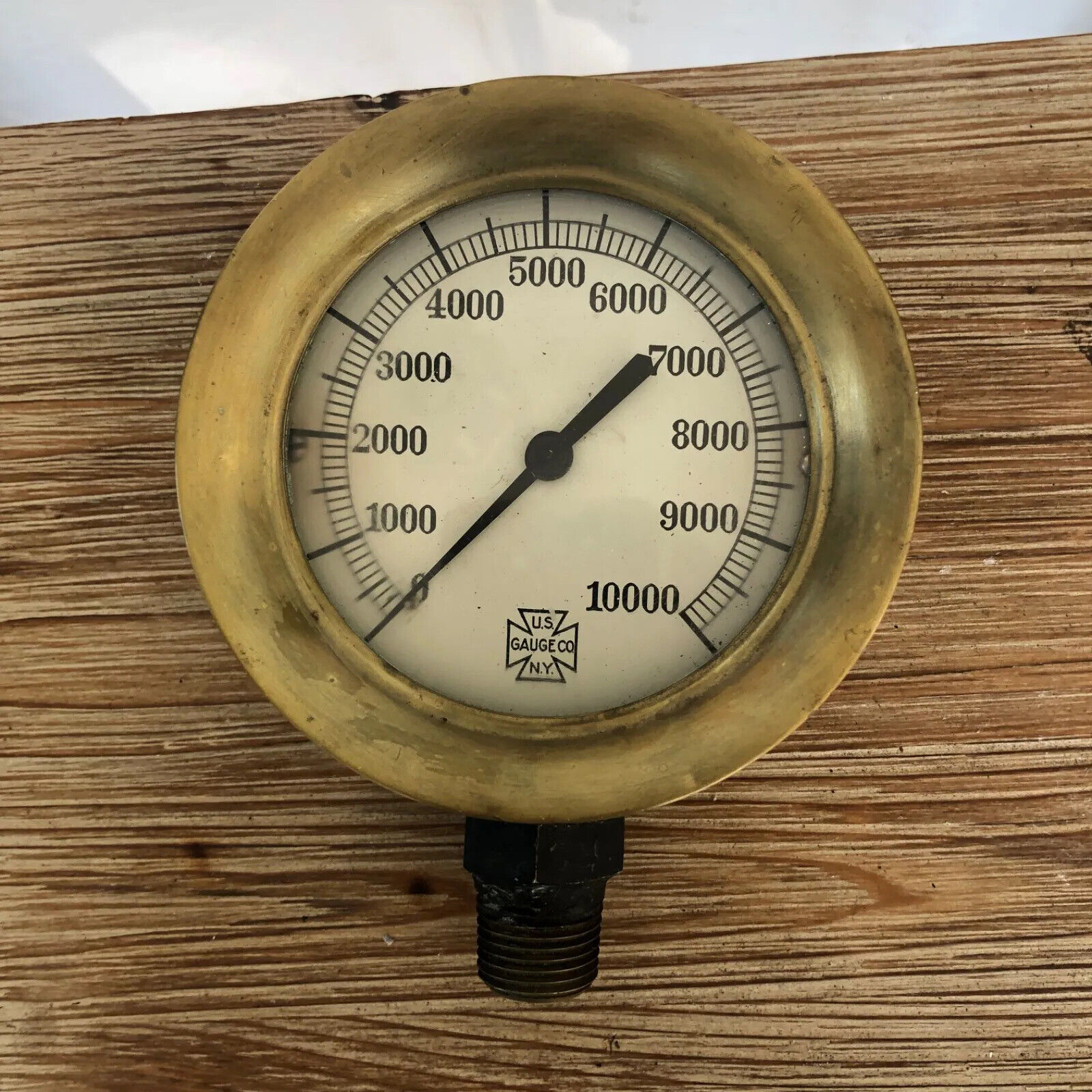The image showcases an antique pressure gauge with a worn, bronze or golden-brown circular frame. The gauge, which is affixed to a wooden surface, is graduated from 0 to 10,000 in increments of 1,000. At the bottom of the gauge face, there is an iron cross design that reads "US Gauge Company, New York," abbreviated as "US Gauge Co. N.Y." The gauge features a black, pointy arrow indicating a current reading of zero. The device appears to be aged but still functional, with visible signs of wear that add to its antique charm. A black screw beneath the gauge suggests it is securely mounted in its place, though it is unclear what specific pressure it is designed to measure.